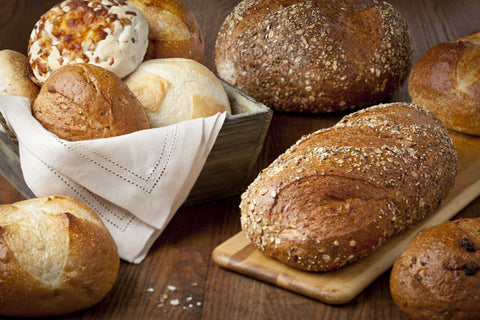The image displays a variety of baked items arranged on a brown table. Prominently, a basket lined with a white cloth napkin contains three distinct rolls: one with a very white appearance and a brown top, another that is uniformly brown, and a third that is primarily white with lighter beige areas. Next to the basket, a darker roll sits alone on the table's surface. On the right side, a wooden cutting board features two loaves of bread: the visible loaf is brown with white speckles on top, while only the end of the second loaf is discernible. The assortment of bread, totaling about ten pieces, suggests a setting akin to a restaurant, given the quantity and presentation. There is also a noted pinch of salt on the table, possibly hinting at a seasoning detail or a culinary touch.